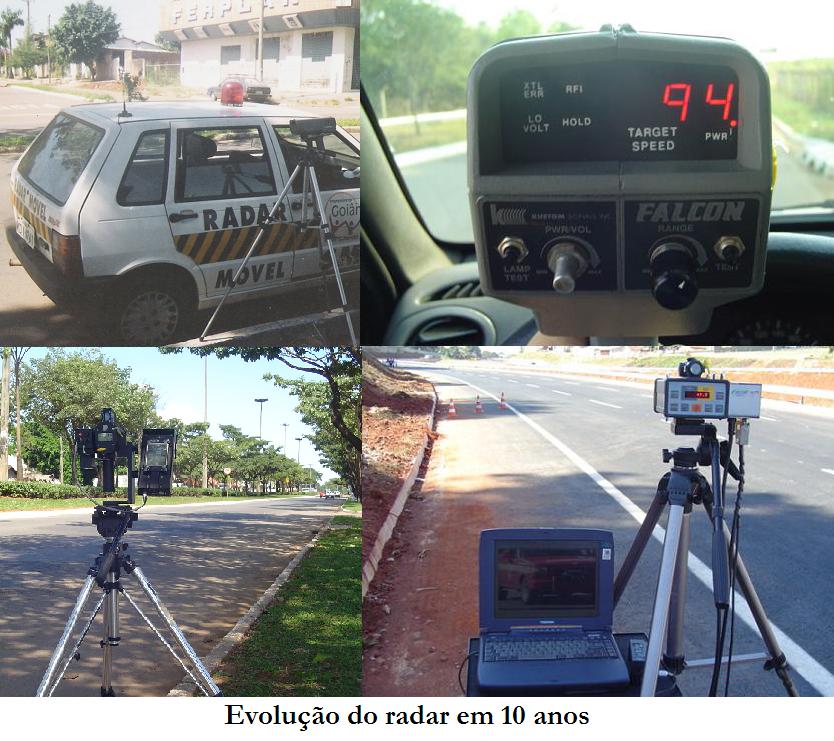In a picturesque Spanish-speaking country, an intriguing setup of radar equipment is featured across four photographs. The first image showcases a white police car with bold yellow and black stripes and the label "Radar Móvel" on its side, parked against a curb amidst modest, single-story buildings. Adjacent to the car, a radar device, perched on a tripod, diligently monitors traffic.

The second photograph captures the dashboard interior of the vehicle, dominated by a Falcon-branded radar gun. The gun displays a target speed of 94, indicated alongside various operational signals: XTL, ERR, RFI, low voltage, and hold. The power and range buttons of the device are illuminated, denoting active status.

Moving to the third image, the same radar gun is seen pointing down a green-laden street from a window, indicating its functional reach beyond the confines of the car. Alongside the road is a green embankment, further emphasizing a thoroughfare under vigilant surveillance.

The final photograph focuses on another radar setup, this time connected to a computer, stationed on the roadside. Three traffic cones mark the vicinity, while text at the bottom, "Evolução do Radar em 10 Anos," highlights advancements in speed monitoring technology over the past decade. This comprehensive depiction melds historical and technological narratives into a coherent observation of traffic enforcement in a quaint locale.